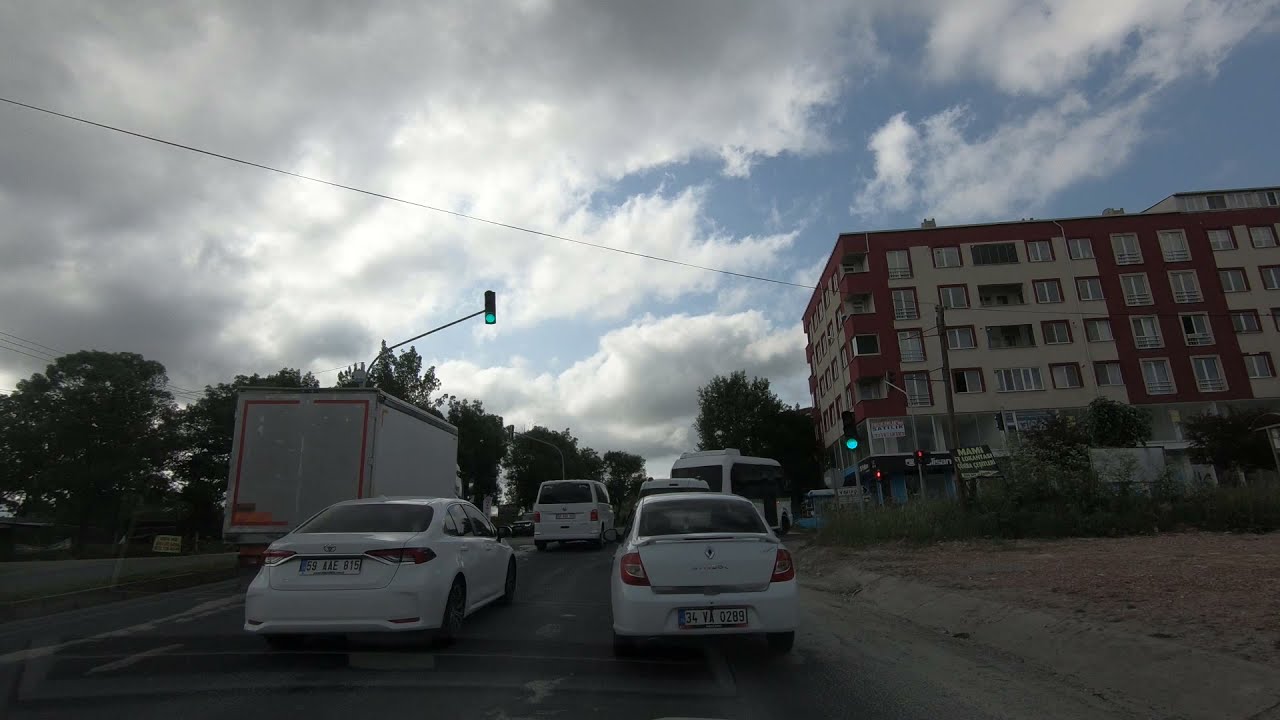The photo captures a bustling urban street scene on a daytime with partly cloudy blue skies. Central to the image is a three-lane road filled with vehicles: a box truck in the left lane, a white van, and a white sedan in the middle lane, along with another white compact car directly in front. There are visible license plates on two of the white cars; one reads 34VA0289, and the other 59AAE815. A bus, potentially making a right turn, is also seen up ahead near the green traffic light.

On the right side of the image, a patch of dirt with weeds growing at the edges separates the road from a brown, five or six-story building with numerous windows. Some of the windows of this red-brick building are open, suggesting it might be an apartment complex. Trees line the street, adding a touch of green to the scene. The sky features a mix of fluffy, white clouds and some gray patches, indicating a possible impending rain. A green stoplight and a sign positioned to the right of it are also part of the composition.